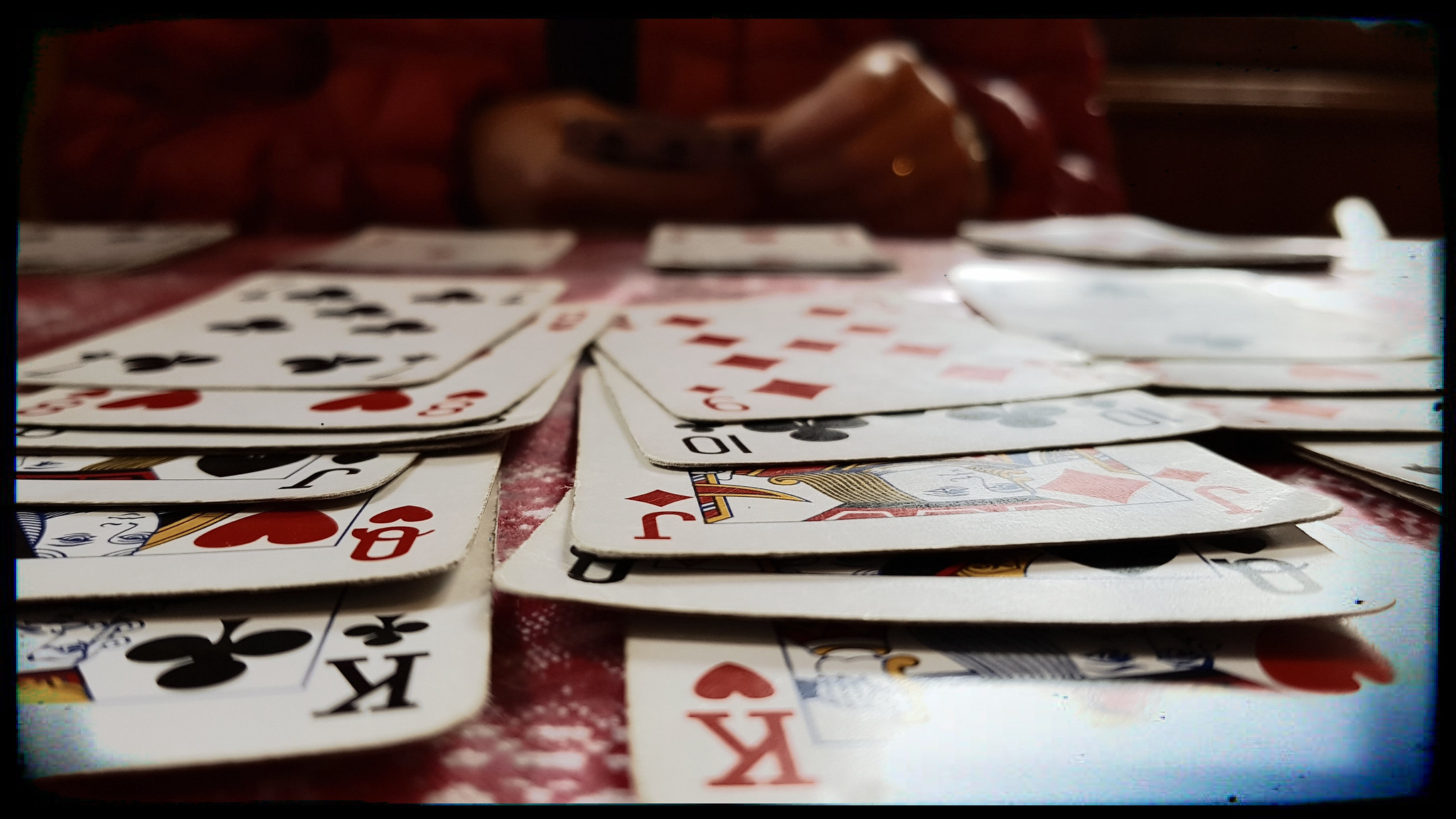This photograph captures a close-up, eye-level view of a deck of cards meticulously arranged on a tabletop, indicative of a Solitaire game in progress. The camera angle is so low that it almost seems as if the table itself is observing the scene. In the foreground, several cards are prominently displayed: a king, queen, jack, and ten, all alternating in color from red to black. Specifically, the layout begins with a King of Hearts on the right and a King of Clubs on the left. 

In the lower part of the image, there are four cards placed side by side, hinting at the foundational aces typically lined up to organize cards from ace to king in Solitaire. In the background, a person in a vibrant red coat is also visible. Both of their hands rest on the table, clutching a few cards, with a noticeable ring adorning the ring finger of their left hand, adding a touch of personal detail to the scene. This meticulously framed shot not only highlights the intricacies of the game but also offers a glimpse into the person engaged in the leisure activity.